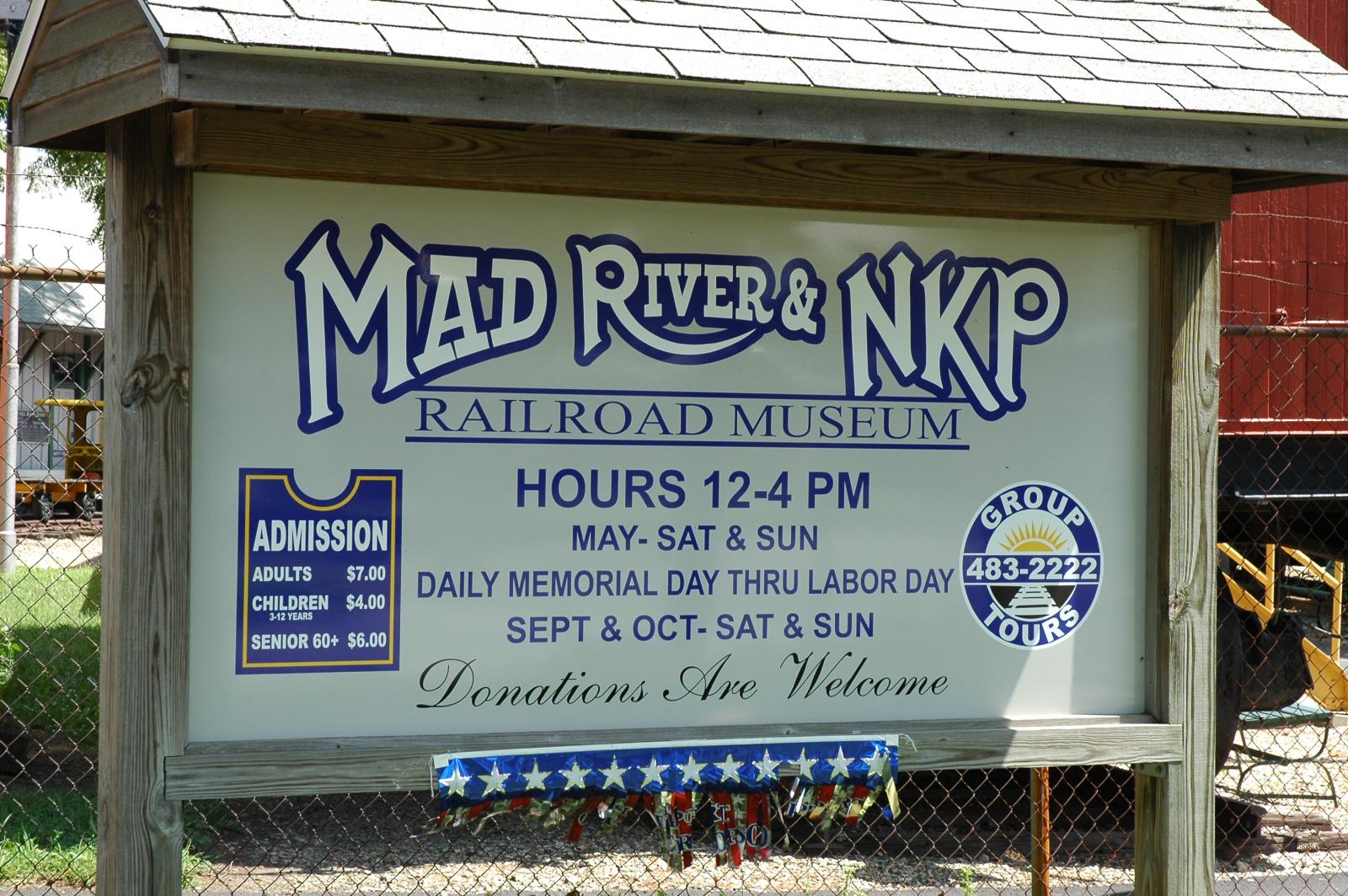This is an outdoor photograph of a well-detailed sign for the Mad River and NKP Railroad Museum. The sign, made of grey wood, is protected by a small roof with white shingles and is mounted between two wooden poles. The center of the sign features large block letters with a white and blue border that read "MAD River and NKP" on a grey background. Below that, the text "Railroad Museum" is prominently displayed in blue.

The operational hours are clearly listed: "Hours 12 to 4 p.m. May, Saturday and Sunday. Daily Memorial Day through Labor Day. September and October, Saturday and Sunday." Beneath this, in black italics, the sign states that "Donations are welcome."

The left side of the sign provides admission details in white text on a blue background: "Admission: Adults $7, Children (3-12 years) $4, Seniors (60+) $6." On the right side is a circle featuring an image of a sunshine and railroad tracks, along with the text "Group Tours: 483-222." Below the main information is a blue banner adorned with white stars. In the background, there is a metal fence and what looks like a miniature train against a station house with red wooden slats arranged vertically.